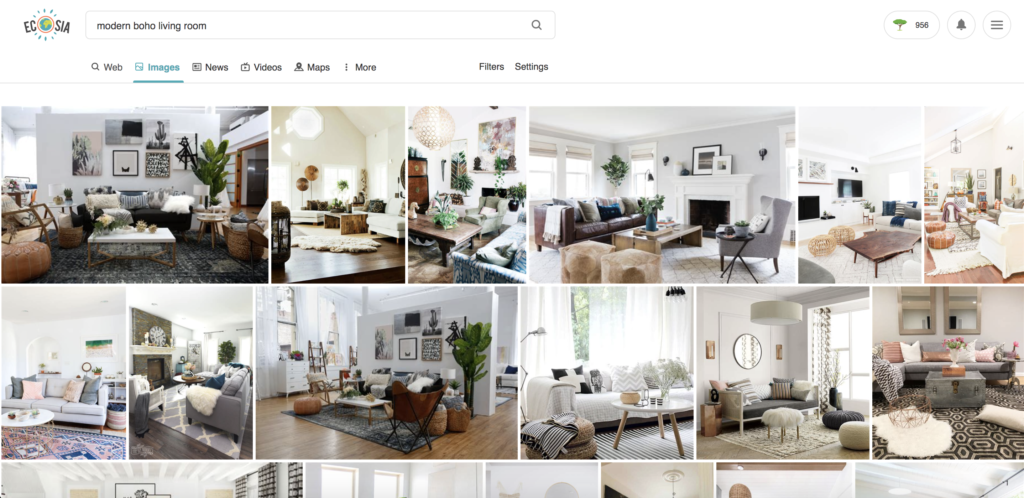Echocia Modern Bohemian Living Room: The images showcase a stylish living space characterized by its elegant blends of modern and bohemian design elements. The main living room features a sleek gray floor and pristine white walls adorned with vibrant paintings. Green plants add a touch of nature, while a cozy fireplace serves as a focal point. Comfortable brown footstools and a central white table complete the seating area. Adjacent to this space is another room, continuing the theme with white walls decorated with artistic hangings and paintings. This room includes a plush white couch, a sturdy brown table, and a large green rug that adds warmth and color to the setting. The combination of modern fixtures and bohemian touches creates a harmonious and inviting atmosphere.